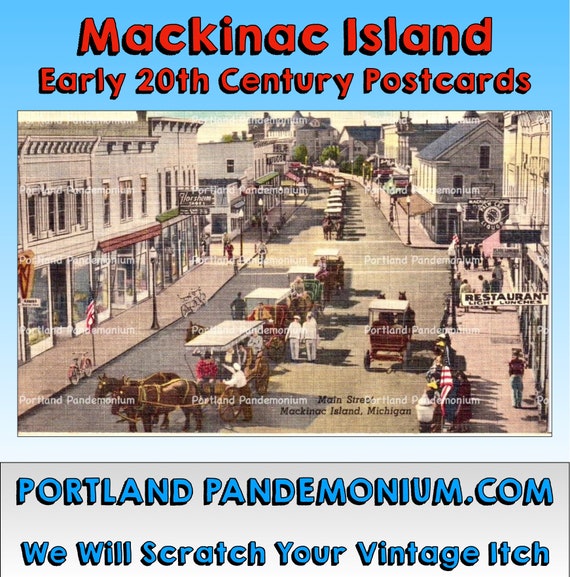This detailed illustration captures a vintage postcard of Mackinac Island dating back to the early 20th century, bordered by a light blue frame with the title "Mackinac Island, Early 20th Century Postcards" written in red at the top. The depiction reveals a bustling Main Street lined with light gray, old-style buildings adorned with American flags. The scene showcases numerous horse-drawn carriages transporting cabbages with white tops, and pedestrians walking along both sides of the street. Among the details, some carriages and seats are rendered in different colors, including green and red, with wooden accents. Prominent storefront signs, including a restaurant and a liquor store, stand out amidst the muted color palette. Two men in white uniforms are positioned near the middle of the street scene, adding to the historical ambiance. A watermark reading "Portland Pandemonium" is present, alongside a tagline at the bottom of the postcard: "Main Street, Mackinac Island, Michigan" and "PortlandPandemonium.com. We will scratch your vintage itch."